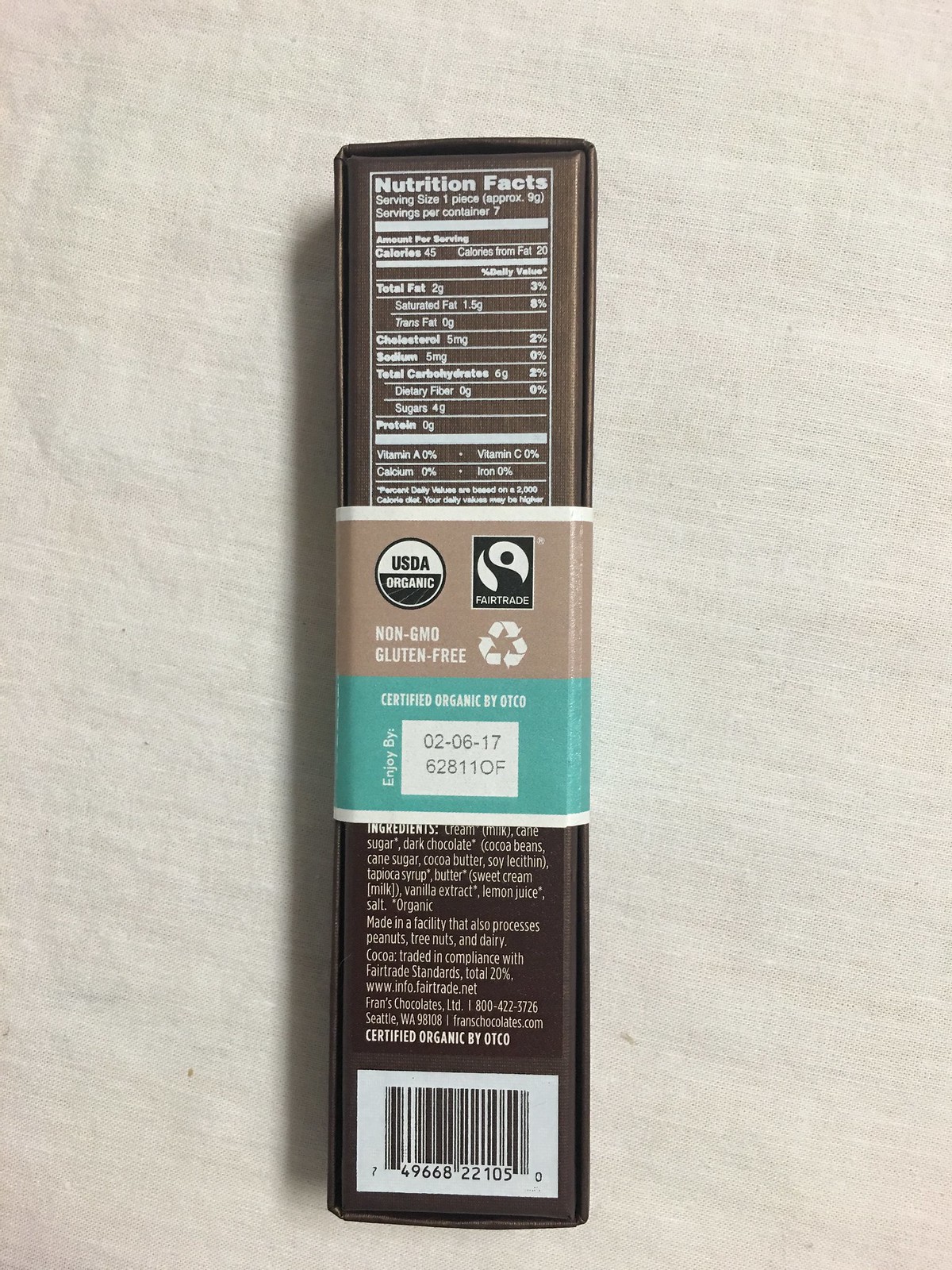The image depicts a vertically rectangular object set against an off-white background. The main focus is a narrow, vertically rectangular box, likely a food or snack package displayed from the back. The box has a dark brown color and features a wrapper around its midsection. The upper half of the wrapper has a light tan to light brown background, while the lower half is teal.

On the wrapper, several emblems and labels are visible, including the USDA Organic emblem and the Fair Trade emblem. It also features labels indicating that the product is non-GMO, gluten-free, and certified organic, accompanied by the OTC logo. There is also an expiration date marked as "2-6-17" and a serial or manufacturer's number.

Above the wrapper, the box displays a nutritional facts panel in white against the dark brown background. Below the wrapper, a list of ingredients is also printed in white. At the very bottom of the box, there is a white section containing a black UPC code.